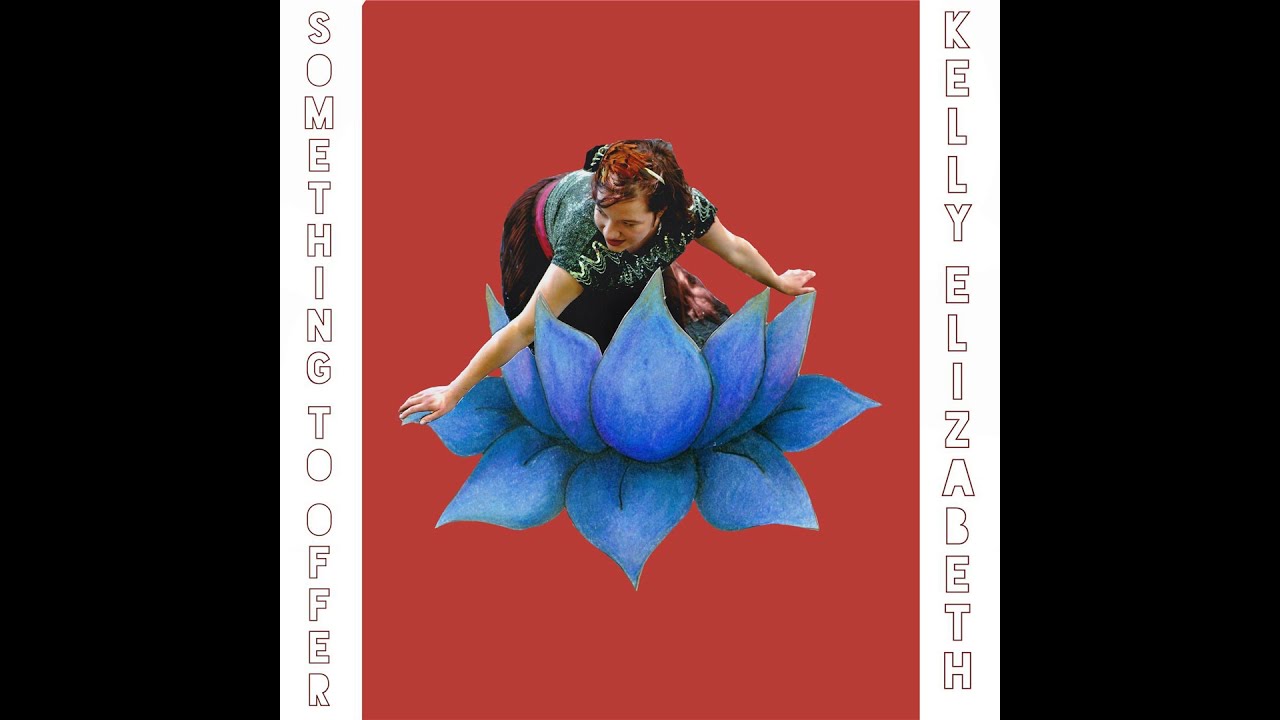The image is a color photograph of a suggested album cover set against a black background with thick black outlines on either side. At the center is a dark red rectangular background. Vertically aligned along the left edge of the red rectangle are the words "Something to Offer" in an outlined black box font filled with white, with unique O's and R's that lack inner detailing. Similarly, on the right edge, the text "Kelly Elizabeth" appears in the same font style.

In the middle of the red rectangle is a large blue flower, its bottom petals flat and top petals arching upwards. Superimposed at the center of the flower is a photographic image of a woman in her 20s with red curly hair and wearing a black shirt. She is bent over at the waist, her arms extended to touch the petals of the flower. The style combines photographic realism and illustrative art, delivering a modern, mixed-media aesthetic.